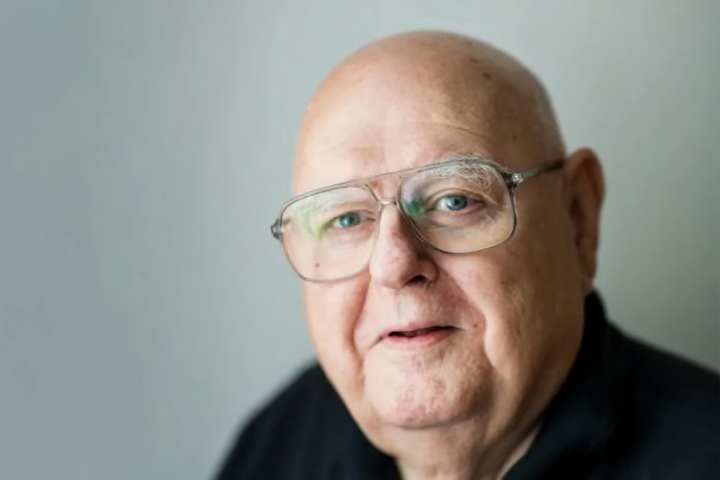The photo features an older, bald gentleman, estimated to be between 60 and 80 years old, who is slightly overweight. He has big, white eyebrows and blue eyes that convey a cheerful expression. His face is characterized by a double chin, puffy cheeks, and a few wrinkles on his forehead. He dons large, aviator-style glasses with pale grey frames and is dressed in a black shirt. The image is taken from a slight side angle, showing the left side of his face and ear. The background is a pale greyish blue, and the man has a faint smirk as if he's about to say something.